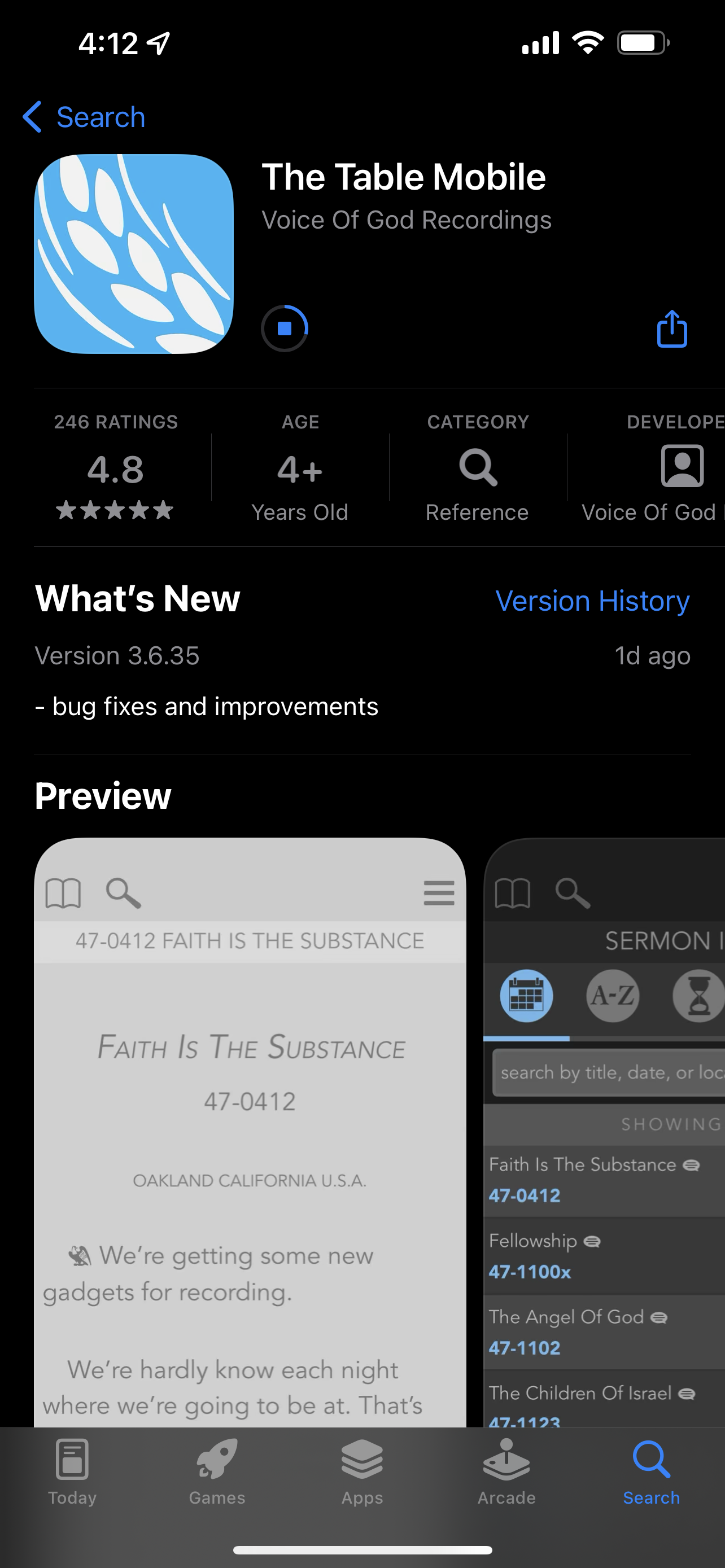Detailed Descriptive Caption:

The screenshot captures various interface elements at the top of the image, starting with a status bar displaying the time "4:12" in white, accompanied by icons for an airplane mode (depicted by a paper airplane), Wi-Fi, and battery level. 

Below this is a blue header with a back arrow and a "Search" function. Further down, there is a blue and white square featuring a design with wheat-like elements and wavy lines. Within this square, in white text, it reads, "The Table Mobile Voice of God Recordings," accompanied by a blue play icon.

Additionally, there's a section showing user ratings: "246 ratings" with an average of "4.8 stars." It also includes the information that the app is suitable for ages four years and older and falls under the "Reference" category, developed by "Voice of God." A small square with a person icon is also visible here.

This is followed by the "What's New" section, detailing the latest version (3.6.35) with "bug fixes and improvements" and showing the update history as "one day ago." Below this are preview windows on a gray background featuring a book icon and magnifying glass icon. The text reads "47… 04… 12 Faith is the Substance, Oakland, California, USA." Partially visible text mentions recording gadgets.

Further down is a gray box containing a blue calendar icon, an A-Z icon, an hourglass icon, and a search functionality, displaying topics like "Faith as a Substance," "Fellowship," "The Angel of God," and "Children of Israel."

At the bottom of the screenshot are several icons and categories: a gray "Today" news icon, a gray rocket icon labeled "Games," a gray square icon tagged "Apps," and a joystick icon named "Arcade." The bottom of the screen features a blue magnifying glass icon next to a white line.